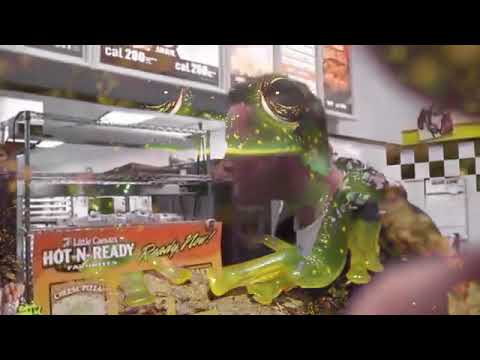The image depicts a man inside what appears to be a fast-food restaurant, identifiable by the menu visible at the top of the screen. The overall picture has black borders at the top and bottom, each about an inch wide. A box in the lower part of the screen is labeled "Little Caesars Hot and Ready." The man is of light skin complexion with dark short hair, and the background shows a checkered pattern on the wall along with various signs. His face is obscured by a green, sparkly substance, which could either be a reflection or something drawn over the photo, adding to the distortion. The man seems to be interacting with a microwave. The overall scene feels somewhat disjointed and discombobulated due to the overlay and reflections.